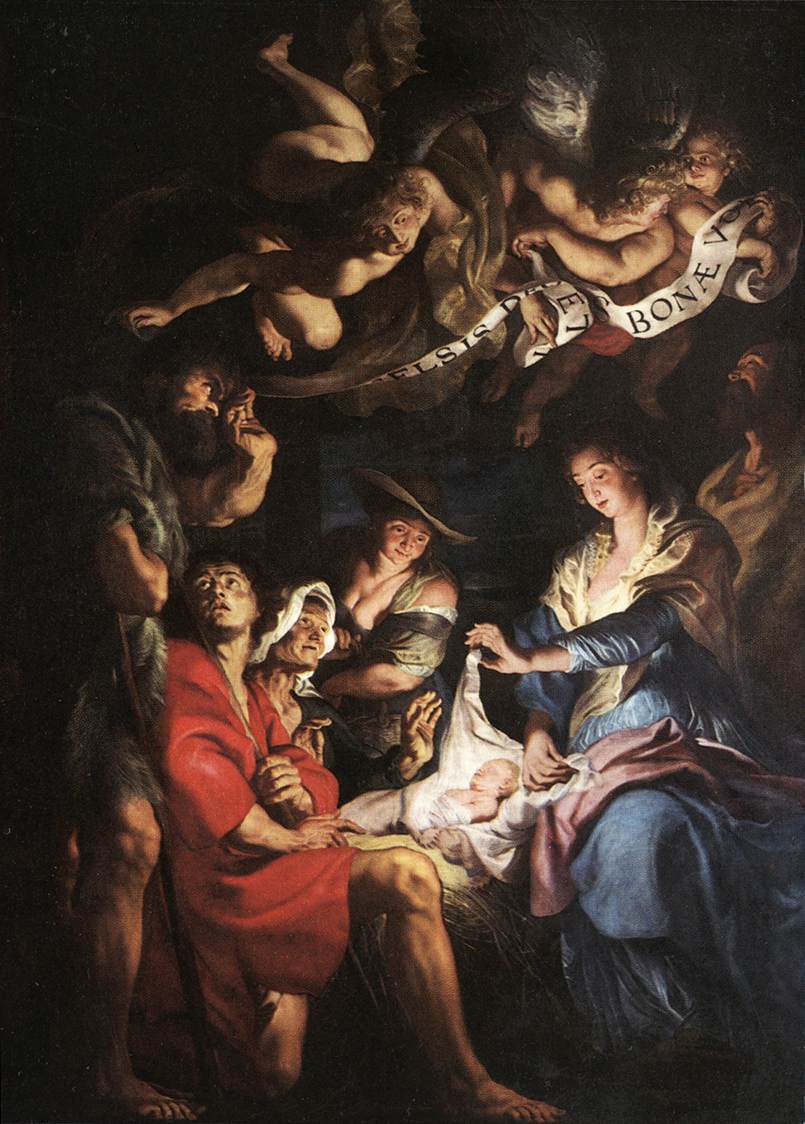This detailed painting, likely an oil painting, is an indoor religious scene depicting the birth of a baby, who appears to be the baby Jesus. The central focus is the baby dressed in white clothing and lying on a white cloth, emanating a bright light that illuminates the entire scene.

Around the baby, various figures are gathered, their expressions and postures reflecting reverence and adoration. To the right and slightly above the baby, a woman in a blue dress—possibly the Virgin Mary—is holding up the baby blanket, gently lifting its corners. She has brown hair and wears a serene expression. Behind the baby sits a large woman in a green dress and hat; she looks down at the infant with tenderness. 

To the left of the baby, a man in a red robe is kneeling, one knee on the ground, and looking up toward another man standing beside him. This standing man, possibly a shepherd, has a beard and wears gray garments. Another figure, an older woman in a gray dress with a hat, has noticeable cleavage and stands in the background gazing down at the baby.

Above this poignant scene, two angels or cherubs are depicted flying and holding a white banner. The banner contains partially readable Latin or Greek lettering, including the letters B-O-N-A-E.

The artistry of the painting emphasizes the sacredness and divinity of the moment, with light radiating from the baby creating a halo effect that highlights the holiness of the newborn Jesus surrounded by adoring figures and celestial beings.